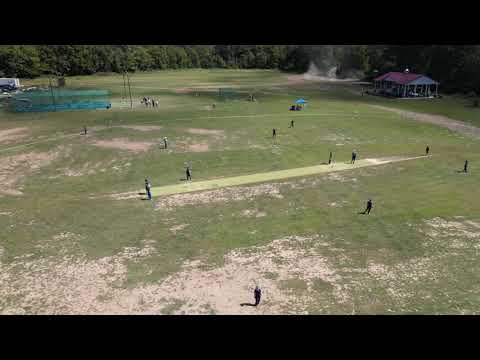This photograph, framed by solid black bands at the top and bottom, captures a vibrant park-like field on a sunny day. The field itself is a patchwork of ragged, late-summer grass interspersed with bald spots and dirt patches. Scattered across the terrain, several individuals are strategically positioned, suggesting an informal game akin to baseball or cricket, though no distinct equipment or markings define it as such. Prominently located in the background is an open-sided pavilion with a red roof, flanked by picnic tables and an outdoor setting featuring a blue umbrella with people underneath. Further into the background, on the left, some green fencing partly encloses a parking area, where at least one car can be spotted. To the right, a house with a triangular red roof stands near a backdrop of dense green trees, completing the serene yet lively scene.